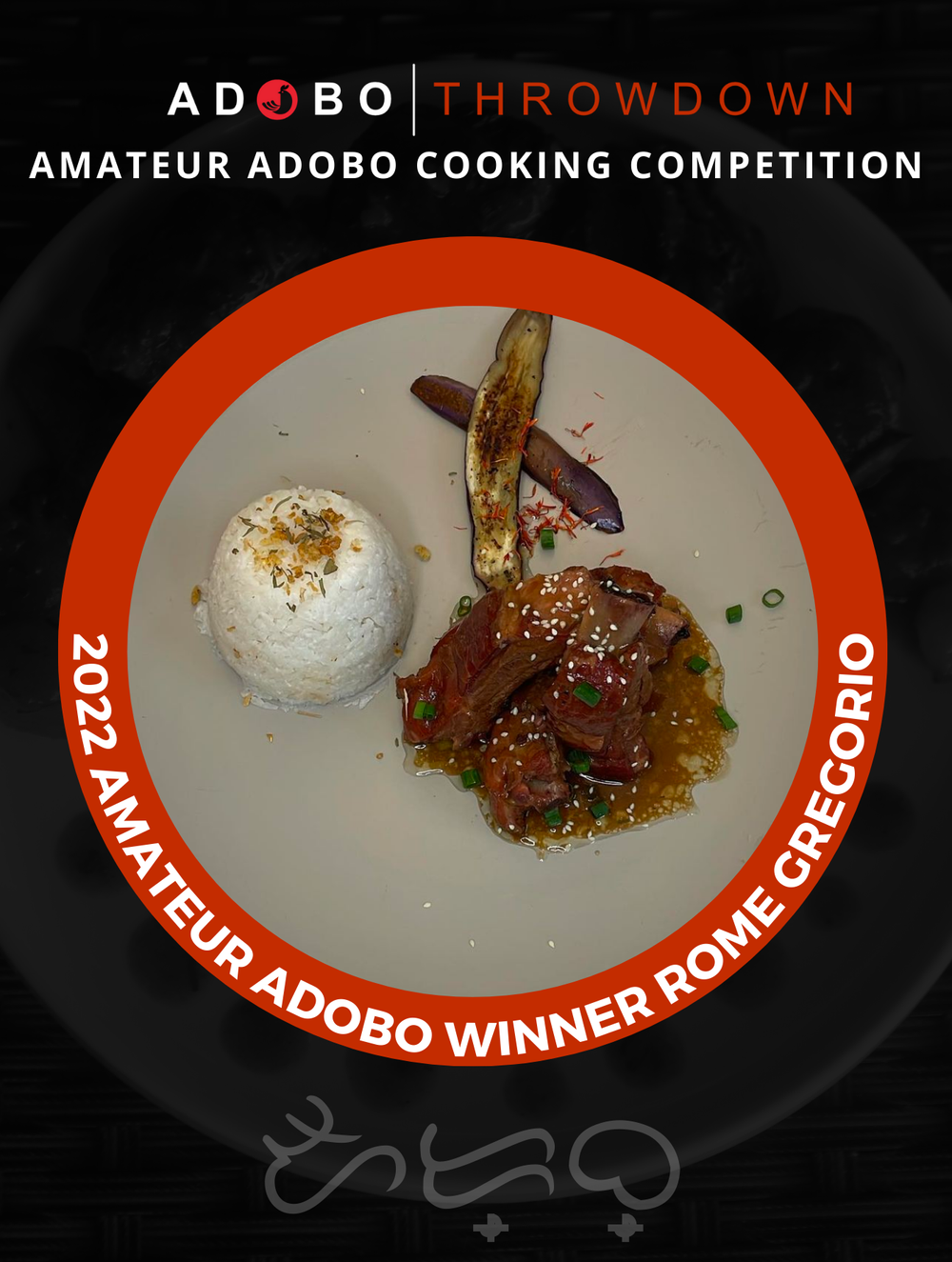The image showcases a meticulously plated food dish prominently placed in the center on a gray plate or surface, set against a black background. At the top of the image, bold white letters announce, "Adobo Throwdown, Amateur Adobo Cooking Competition." The focal dish is encircled by a red border, highlighting its significance as the "2022 Amateur Adobo Winner." Alongside this accolade, the name "Rome Gregorio" is clearly labeled. The dish itself features a perfectly scooped mound of white rice on the left, resembling the shape created by an ice cream scooper. To its right, there's an intricate presentation of adobo, a savory Filipino delicacy, which includes tender orange meat pieces delicately stir-fried with sesame seeds, alongside chopped onions and eggplant slices. Below the descriptive text, a distinguishable logo, appearing to be a dragon or bird, intricately forms curving letters, adding an artistic touch to the presentation.